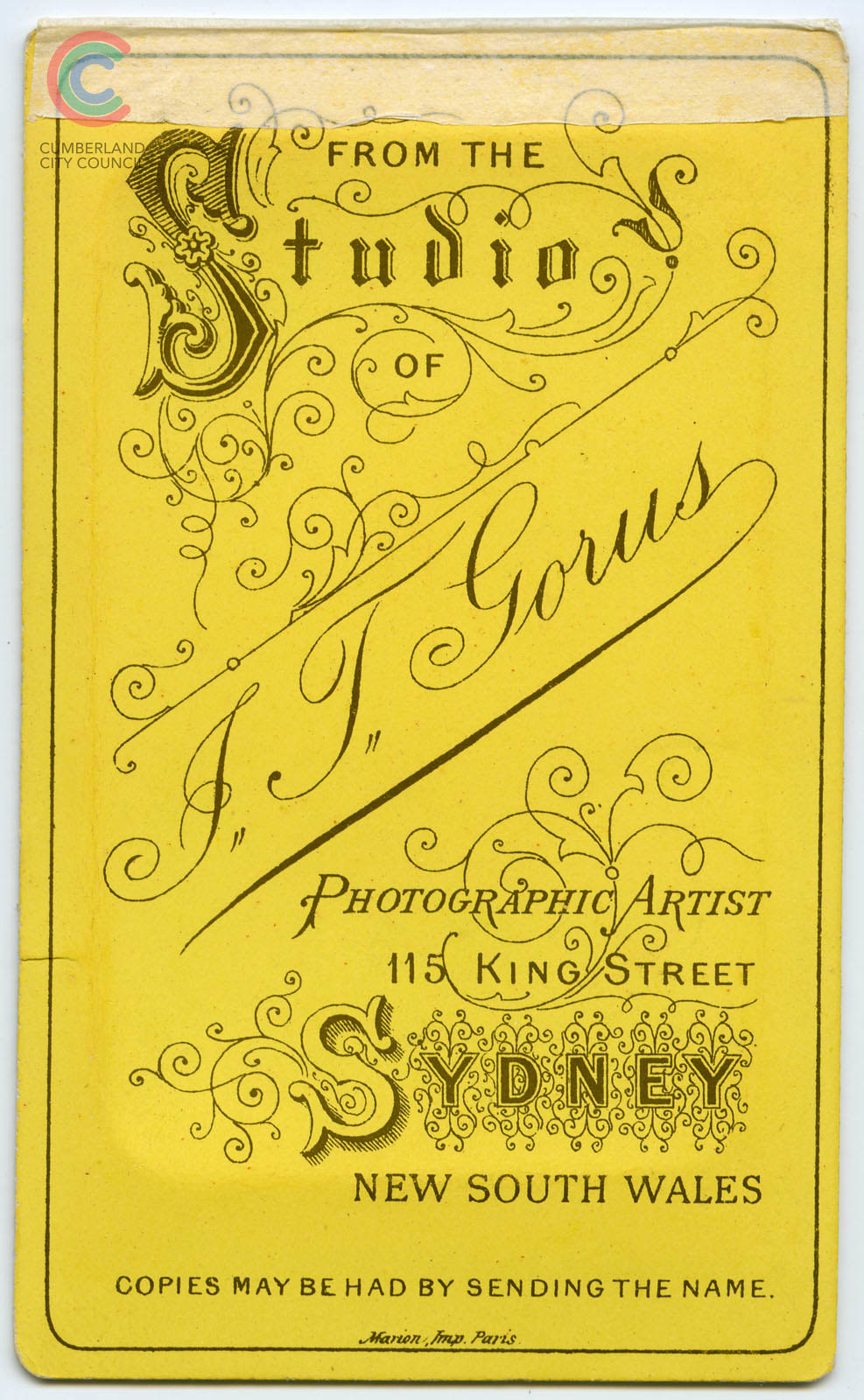The image depicts the front cover of a vintage book or poster, seemingly protected by a plastic or tin layer. The dominant color is yellow, with intricate black scroll work and a thin black border framing the rectangular, portrait-oriented layout. A strip of masking tape is affixed to the upper edge, adding to the aged appearance. At the top right corner, there is a vibrant logo featuring three concentric "C"s in red, green, and blue, labeled as the emblem of Cumberland City Council.

The title reads "From the Studio of J.T. Goris, Photographic Artist, 115 King Street, Sydney, New South Wales" in an artistic and stylized black font. Below this, a footnote states, "Copies may be had by sending the name." At the bottom of the design, a delicate signature is present alongside the words "Marion in Paris." Overall, the intricate patterns and old-fashioned style of the typography suggest this cover is likely from a publication dating back around a hundred years.